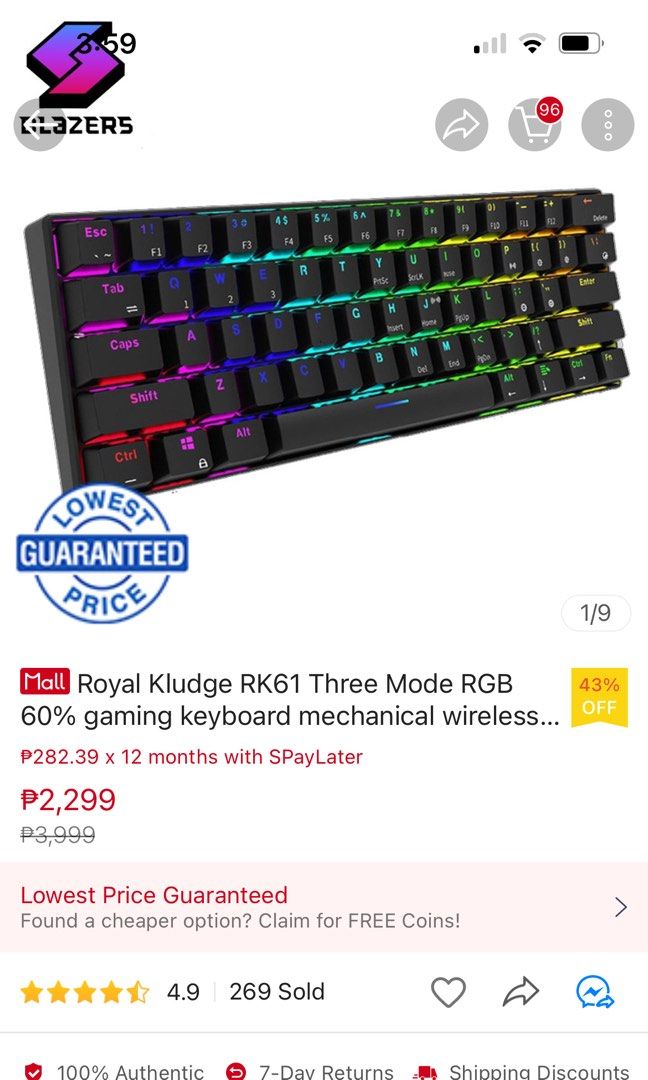This screenshot captures a product listing for a keyboard on a smartphone. The time displayed on the top left is 3:59, though it is somewhat obscured by the background. The battery icon on the top right indicates approximately 80% charge. The top-left corner features the brand name "Blazers," but the letters "B," "L," and "A" are partially hidden behind a back arrow overlay. The interface also includes a share button and a cart icon on the top right, showing 96 items currently in the user's cart. Additionally, there is a three-dot menu for more options.

The keyboard showcased is predominantly black with vibrant, multi-colored backlighting that gives it a dynamic, glowing appearance. The lights include shades of red, pink, blue, green, light blue, yellow, and orange, creating an eye-catching effect. The model of the keyboard is identified as the "Royal Kludge RK61," and a label at the bottom left of the product image assures the "Lowest Guaranteed Price."